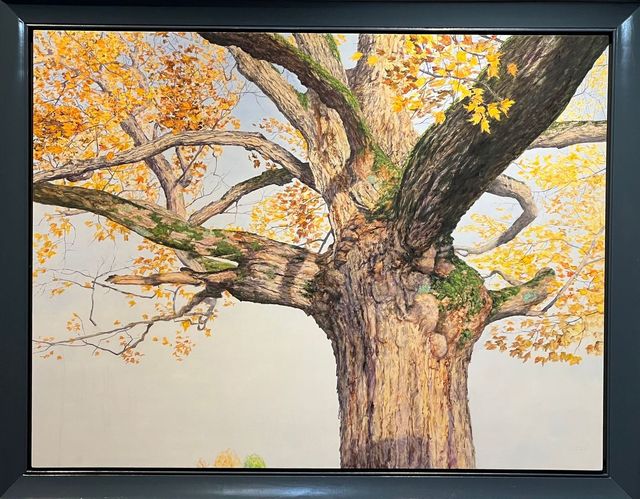This is a very detailed pencil sketch of a tree, framed within a photorealistic blue frame. The artwork captures a close-up view from the base of a thick, gnarled tree trunk, accented with a prominent burl. The perspective makes it feel as though you're looking up through the tree, with branches extending in various directions, some covered in green moss. A large branch juts off to the left while another curves towards the top right corner. Smaller branches seem to emerge randomly, adorned with numerous jagged-edged, yellow leaves reminiscent of maple leaves, indicating either the onset of fall or early spring. The tree itself is drawn in light brown tones, conveying a healthy, vibrant impression, despite the gray, overcast sky in the background. The sky, mostly obscured by the branches and leaves, has a slight blue tint higher up. Altogether, the detailed and realistic nature of the drawing, combined with the contrasting photorealistic frame, creates a striking and immersive image.